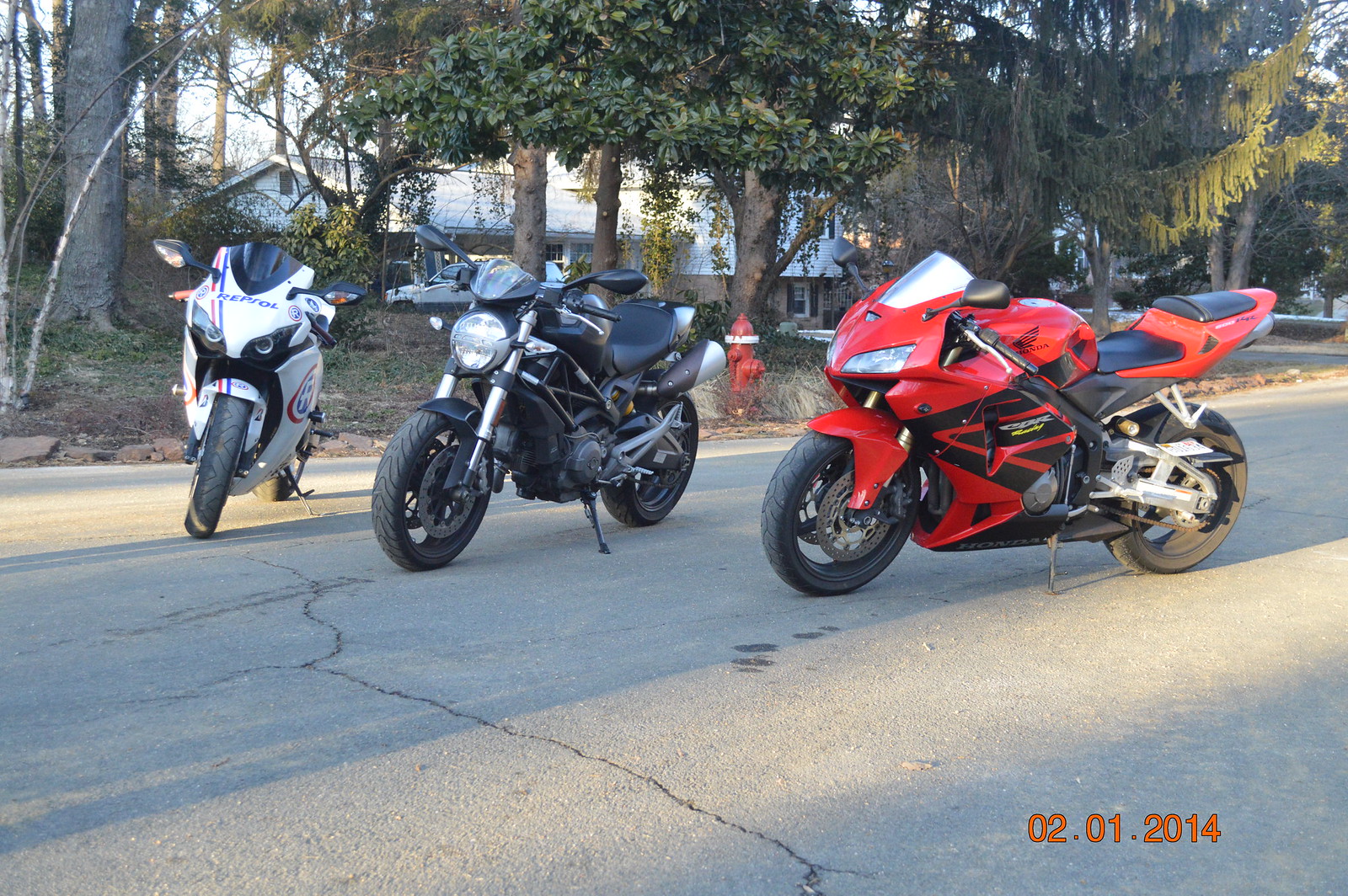This photograph, captured on February 1st, 2014, presents a vibrant outdoor scene featuring three motorcycles parked on an asphalt road. The road, which shows signs of weathering with a prominent crack, is situated in a residential area. In the background, a white, two-story house peeks through a dense cluster of trees adorned with green leaves, suggesting a warm climate even in early February. A red fire hydrant stands prominently amongst the foliage.

The motorcycles are aligned such that their front wheels point towards the lower left-hand corner of the image, with their kickstands down. The motorcycle closest to the viewer on the right is a striking sports bike with red fairings and a black seat. In the center, a sleek, all-black motorcycle stands out with its minimalist design. The motorcycle on the left is white with distinctive blue and red stripes along its left side, positioned at a slight angle towards the camera.

Sunlight filters through the trees, casting dappled shadows and highlights across the scene, adding depth and contrast to the image. Despite the casual, snapshot nature of the photo, it offers a detailed glimpse into a moment where three distinct motorcycles are momentarily at rest.